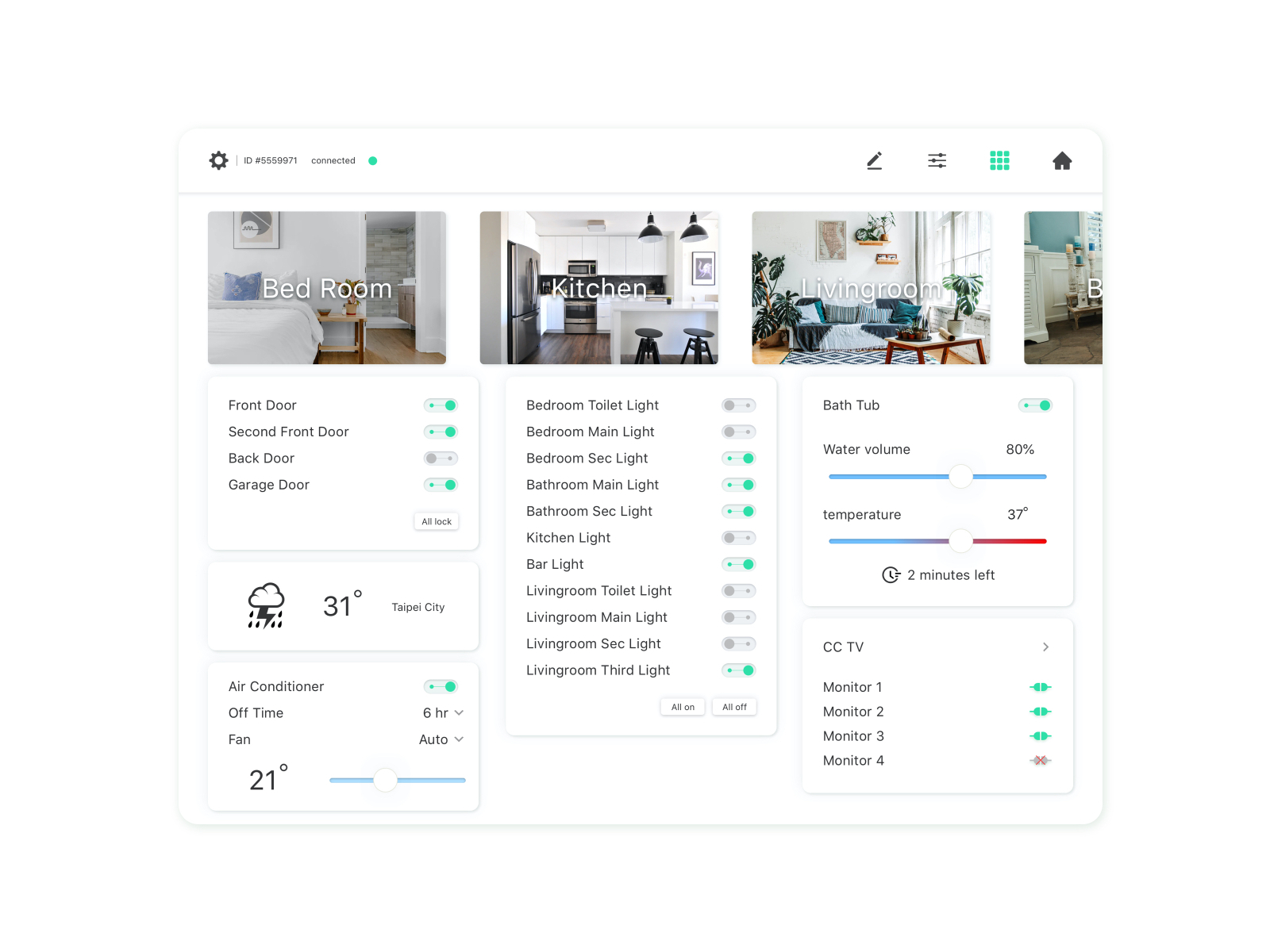An online interface displays three separate photos with detailed information beneath each. 

The first photo depicts a bedroom. Below the image, various home access points are listed: front door, second front door, back door, and garage door. Additionally, a weather icon displays a cloudy sky with lightning and rain, indicating a current temperature of 31 degrees in Tape City. Further down, control information for the air conditioner is shown: it is currently off, set to resume in six hours, with the fan mode set to auto. The room temperature is indicated as 21 degrees.

The second photo showcases a kitchen. Below this image, a comprehensive status of multiple lights across different rooms is presented. The bedroom toilet light, bedroom main light, bedroom secondary light, bathroom main light, bathroom secondary light, and the bar light are all turned on. However, the kitchen light, living room toilet light, living room main light, and living room secondary light are turned off, whereas the living room third light is on.

The third image features a living room.